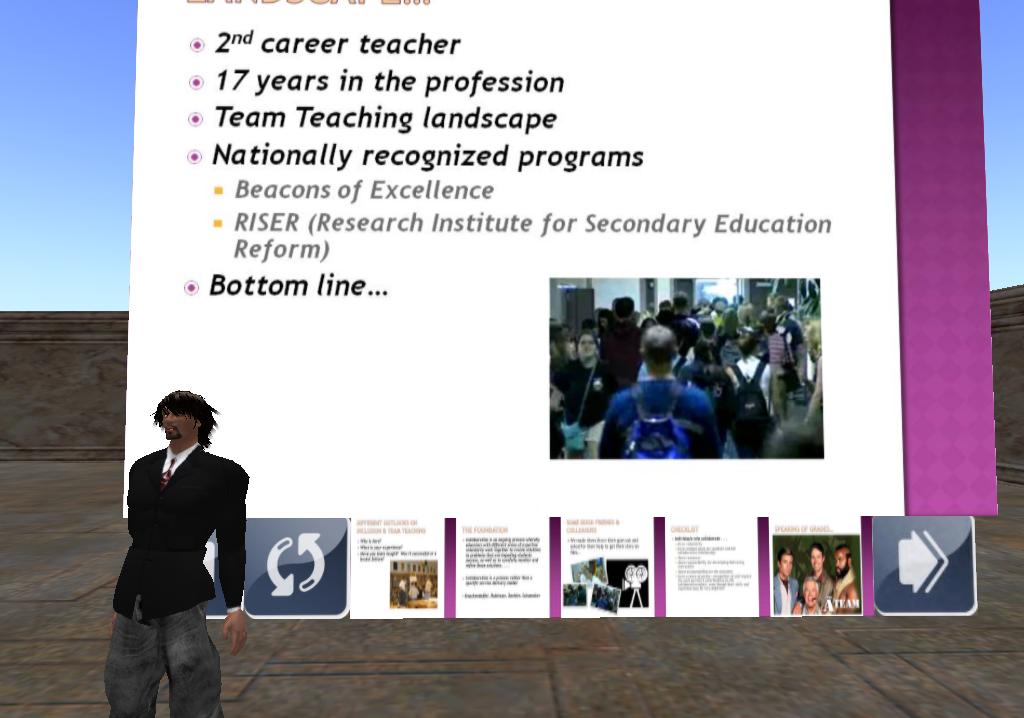The image is a detailed digital screenshot of a three-dimensional space featuring educational content. The setting includes a slate or marble floor and blue walls, with a light blue sky in the background. In the bottom left corner stands a digitally rendered man with long brown hair, a goatee, and mustache. He is dressed in baggy gray pants, a black suit coat, a white shirt, and a red tie. 

The man is positioned in front of a large white screen bordered by a purple stripe on the right side. The screen displays several bullet points in black text, highlighting key phrases such as "second career teacher, 17 years in the profession, team teaching, nationally recognized programs, beacons of excellence, RISER, Research Institute for Secondary Education Reform." Additionally, there is a photograph or video thumbnail showing students walking in a school hallway, some wearing backpacks.

Across the bottom of the screen are several smaller thumbnails that feature text and images, including a notable image of the A-team from the 1980s TV show. These thumbnails likely represent additional pages within the presentation. The detailed and structured layout emphasizes the educational theme conveyed through the presentation.